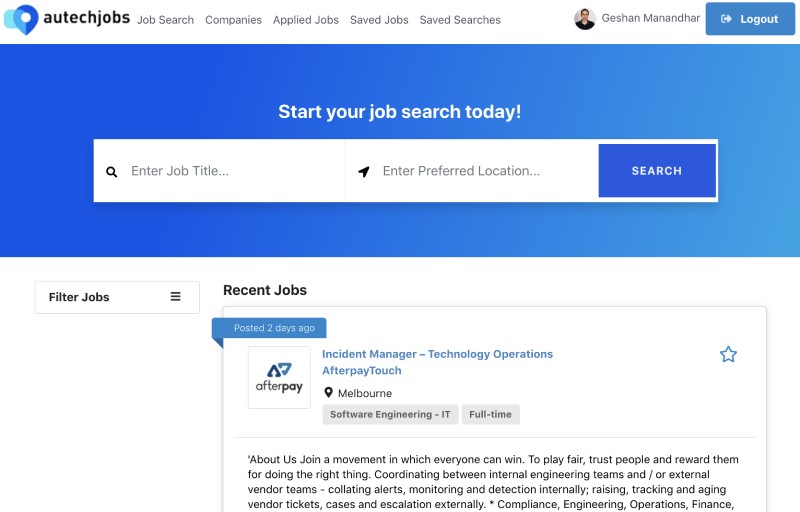**Descriptive Caption:**

The image displays a job posting on a job search website. The top border of the website is white and features a logo in the upper left corner resembling a GPS-style icon, split into light blue on the left and dark blue on the right, with a downward-pointing pinpoint. The navigation bar includes clickable options such as "All Tech Jobs," "AU Tech Jobs," "Job Search," "Companies," "Applied Jobs," "Saved Jobs," and "Saved Searches." 

To the right, there is a profile icon of a person in a black shirt next to the name "Gishan Mannandhar," along with a blue "Logout" button with white text. Below the navigation bar, there is a blue banner that says "Start Your Job Search Today!" featuring input fields for the job title and preferred location, along with a blue "Search" button.

The next section has a white background, with a "Filter Jobs" option followed by a "Recent Jobs" section. This section highlights a job posting made two days ago by Afterpay. It includes Afterpay's logo and lists the position as "Incident Manager, Technology Operations" located in Melbourne under the category "Software Engineering IT" as a full-time role.

The job description briefly outlines the company's values, emphasizing fairness, trust, and rewarding good behavior. The responsibilities include coordinating between internal and external teams, handling alerts, monitoring and detection, managing vendor tickets, and ensuring compliance in engineering operations and finance.